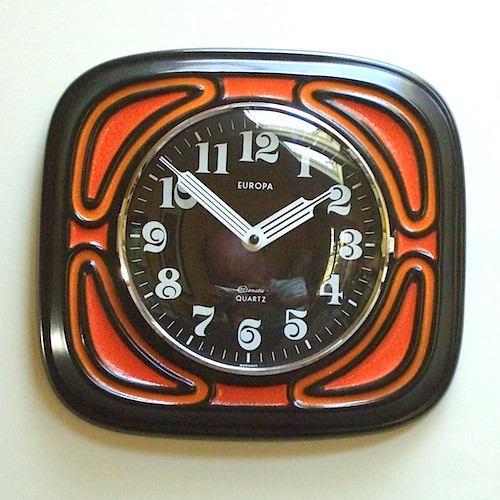This close-up photograph captures a detailed view of a unique clock. The timepiece features a dark brown circular face set into a rounded square casing, which appears to be made of ceramic. The casing is adorned with triangular patterns that have bright orange infills, adding a vibrant touch to the design. The clock face itself displays white numbers and wide white hour and minute hands with long stripes. The word "Europa" is prominently positioned beneath the number 12, while "Quartz" is situated above the number 6 on the clock's white background. There is also a noticeable light reflection on the glass covering the clock face, further enhancing the intricate details of this distinctive timepiece.